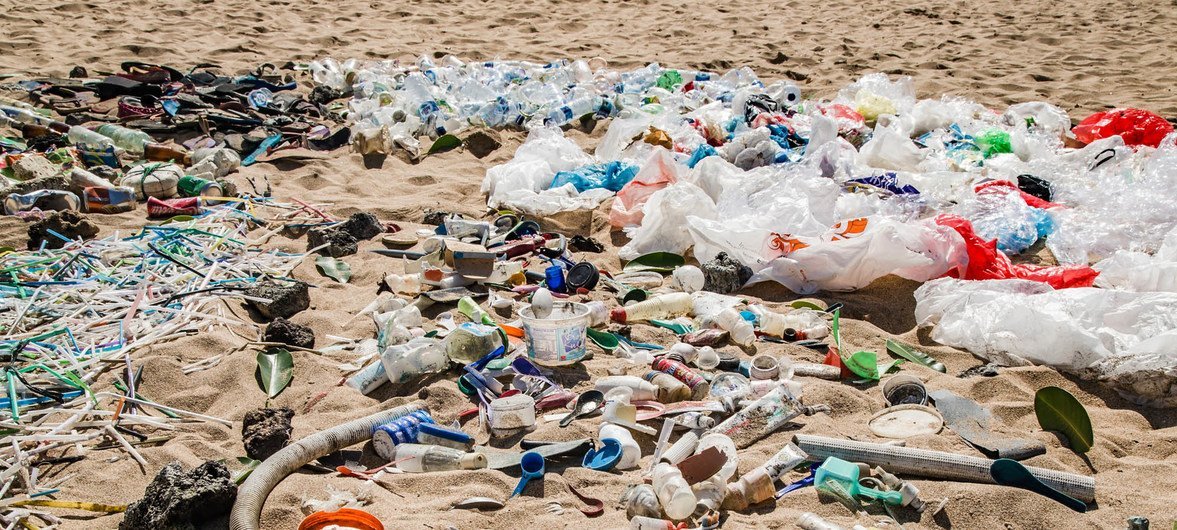In this vivid, daytime beach photograph, an unfortunate scene of oceanic debris is meticulously captured. The sandy beach extends from the foreground to the top of the image, bathed in bright daylight. However, the central focus is on a sizable collection of trash that looks deliberately gathered and organized into sections. The upper portion predominantly features a cluster of plastic bottles, while adjacent to it lies an assortment of plastic bags in shades of white, red, and blue. Below these, a diverse array of debris sprawls across the sand. Among the items are plastic containers, spoons, tubes, toys, mats, straws, and a frisbee. On the left-hand side, small, colorful tubes—blue, green, and yellow—mingle with white plastics and shoes. The middle lower section is strewn with additional plastic waste, including more containers. Interspersed throughout the scene are metal cans, including notable Coke cans, and a peculiar collection of black items, whose nature—be it weapons or electronic devices—remains ambiguous. The landscape hints at human intervention, as the trash appears systematically gathered, highlighting the stark contrast between the natural beauty of the beach and the overwhelming presence of pollution.